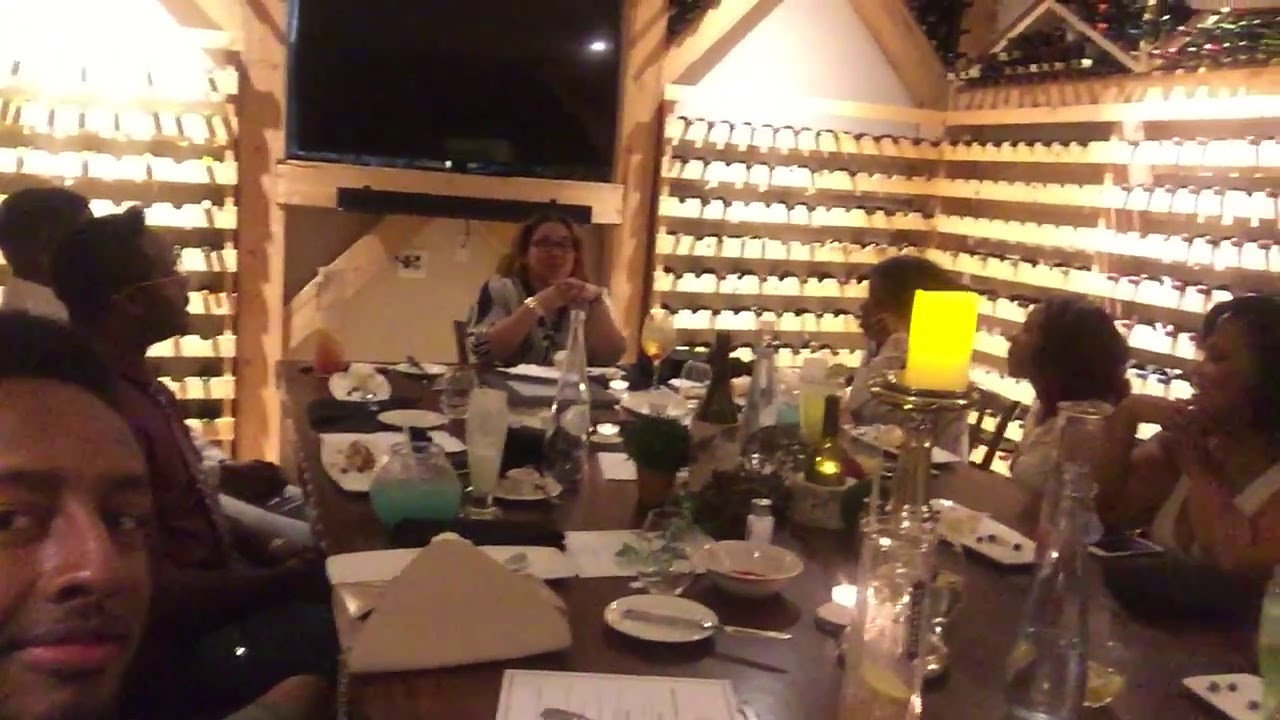In the image, we're inside a brightly lit building characterized by a warm yellowish-orange light. The picture is slightly fuzzy but vivid enough to capture the details of a long table around which people are gathered. On the left side of the table, near the lower left-hand corner, there's a man with brown skin glancing towards the camera, possibly the one taking this selfie. Beside him sit two other men, also focusing their attention to the right side of the table.

On the right side of the table, three women of African descent with brown skin are sitting. They appear engaged and are looking toward the person at the head of the table, who is a woman with light brown skin. She is seated upright, with her elbows on the table and her hands clasped together, central in the photo.

The table is cluttered with typical restaurant items: open glasses that seem to contain wine, plates with remnants of eaten food, salt and pepper shakers, glassware, bowls, and even some papers and candles.

In the background, behind the woman at the head of the table, there’s a large, turned-off TV mounted on the wall. The walls are adorned with multiple shelves, possibly wine racks, holding what could be bottles of wine, adding to the dining atmosphere.